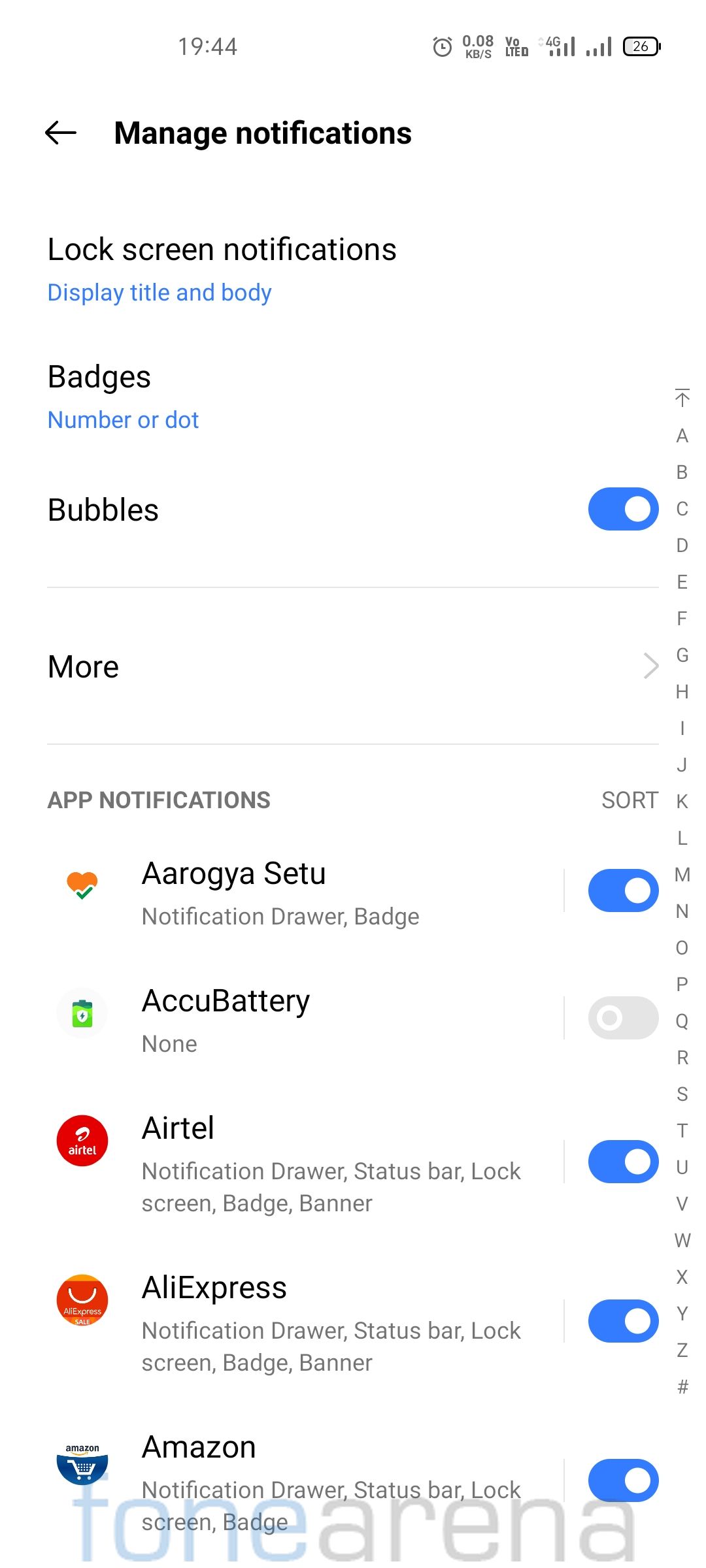This image is a detailed screenshot of the Notifications section of a smartphone. The background is entirely white, creating a clean and unobstructed view of the interface. 

In the upper left corner, the current time is displayed prominently. Moving to the right corner, the status bar includes several icons: a battery icon showing a 26% charge, followed by two internet signal icons. The first internet icon indicates a 4G connection, while the second signifies LTE with "0.08 KB/s" shown below it. There is also an alarm clock icon present in this corner.

Beneath the time on the left side, a bold black left-arrow icon directs the user to "Manage notifications." Following that is a section labeled "Lock notification screen" with an option in blue text to "Display title and body."

Further down, the interface details several notification settings: 
- "Badges" with options to show the number and dot, both articulated in blue text.
- "Bubbles" with a toggle switch on the right side currently activated.

A thin divider line separates these options. Below it, the word "More" is bolded, accompanied by a right-pointing arrow.

In the subsequent section, bold black capitalized text reads "NOTIFICATIONS," aligned with a "Sort" option on the right. Beneath this, five icons are listed vertically, each paired with a descriptive label and an activation toggle. Four out of five of these toggles are enabled, indicated by their blue color and white circle, while the second toggle remains gray and inactive.

Down the right side, from the "Number or dot" section, the labels are alphabetically organized from A to Z, extending through the fourth icon. The interface also features a watermark, displaying "tone" in large blue letters and "arena" in gray text, overlaying the image.